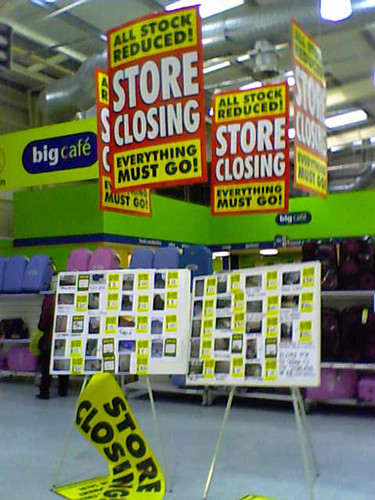The color photograph, a vertical rectangular snapshot, captures the interior of a superstore, likely a Walmart, in the midst of a closing sale. Dominating the upper and middle portions of the image are four large, hanging signs. These signs are red with yellow borders and feature bold black text reading "All Stock Reduced" at the top and "Everything Must Go" at the bottom, with "Store Closing" prominently displayed in large white letters in the center. The industrial ceiling, visible above the signs, showcases an open structure with silver ductwork and large fluorescent lights.

Below the hanging signs, two easels with silver tripod stands hold promotional materials. One yellow sign announcing the store closing has fallen partially to the floor. Alongside these signs are various sale advertisements and images of discounted items. Further into the background, shelves display a variety of suitcases in light blue, pink, black, and purple. To the upper left, a blue sign with a white border and yellow text reads "Big Cafe."

The overall atmosphere of the image is that of a large, somewhat chaotic warehouse environment, typified by grey floors and an assortment of merchandise, highlighting the store's imminent closure and clearance sale.